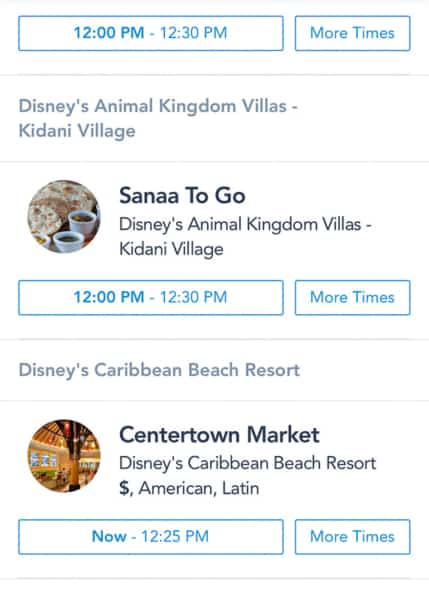This image appears to be a screenshot related to scheduling dining reservations at various Disney resorts. At the top, the time slot from 12:00 PM to 12:30 PM is clearly highlighted, with an adjacent box that allows users to search for additional times. The first entry is for Disney's Animal Kingdom Villas - Kidani Village. This seems to focus on food options, hinted at by small icons of pizza and coffee. Immediately below, another 12:00 PM to 12:30 PM time slot is available for booking.

Following that, there is information on Disney's Caribbean Beach Resort, featuring a thumbnail image of a restaurant, identified as Centertown Market. This market is categorized as offering American and Latin cuisine, denoted by a dollar sign, suggesting it might be affordable. The available time slot for Centertown Market is from now until 12:25 PM, with an option on the right to check for more times.

In summary, the image provides a detailed overview of available dining reservation times and details for specific Disney resorts, including icons and descriptions to aid in selection.